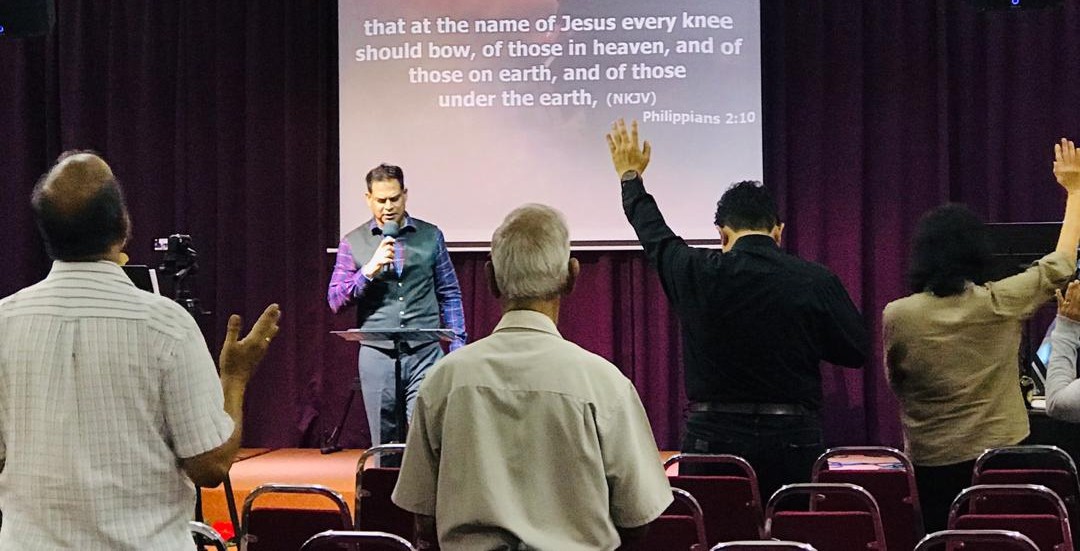The image is a rectangular photograph capturing a church service. At the center, a pastor with short dark hair and light skin stands on a stage behind a small podium. He is wearing a gray vest over a bluish-purple plaid shirt, paired with gray pants, and speaks into a microphone while looking down at his readings. Behind him, a screen projects the text: "that at the name of Jesus every knee should bow, of those in heaven and of those on earth and of those under the earth," followed by "Philippians 2:10" in brackets (NKJV). Dark purple stage curtains frame the backdrop. 

In the audience, visible from behind, several attendees are engaged in the service. A balding man in a short-sleeved white collared shirt stands to the left with his hands raised in a gesture of praise. Beside him, an older gentleman with graying hair, also in a white shirt, stands attentively. To the right, a man dressed in all black and a woman in a tan blouse, both with light skin and dark hair, also stand with their hands raised, palms open and facing upward. Several empty chairs are scattered among the congregation. A video camera on a tripod is positioned in front of the stage, recording the sermon.